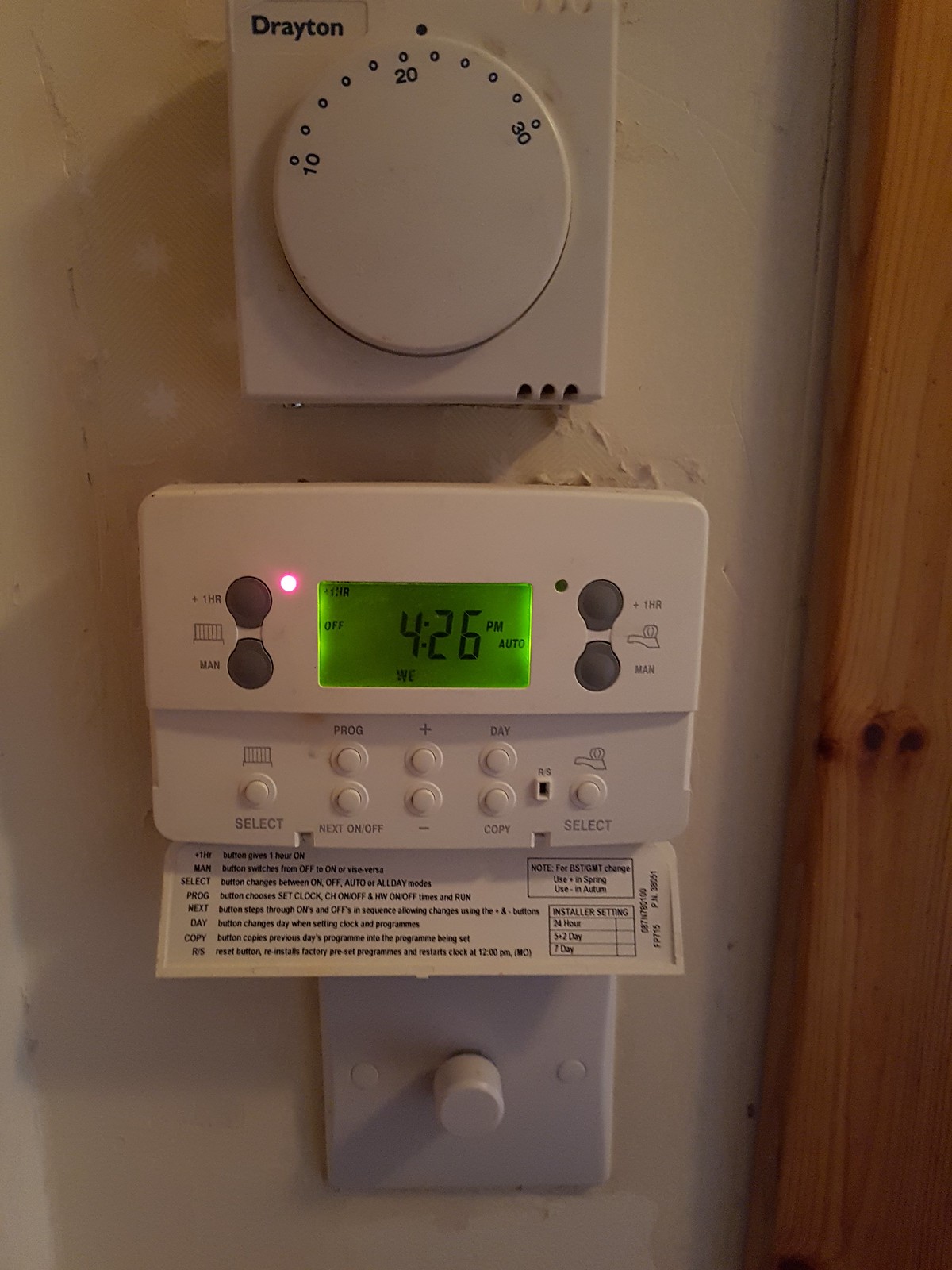The image depicts a portion of an interior wall with a detailed arrangement of various fixtures and elements. On the right side of the wall, there is a piece of maple-colored wood molding, potentially framing a door or window, adorned with three prominent dark knothole markings at its center. At the top of the image, a white plastic box with a raised white dial is visible. This dial features a "10" at the 9 o'clock position and a "30" at the upper right section, surrounded by various dots that extend off-screen. 

Beneath this box, there is an advanced thermostat, characterized by its bottom half that flips open to reveal a panel with controls. The center of the thermostat displays a green, rectangular screen with black digital numbers, illuminated from both left and right sides. To the left of the screen are two gray buttons, the upper one marked by a small white light at the 2 o'clock position. Similarly, on the right side of the screen, there are two gray buttons. 

The open panel section beneath the screen reveals eight smaller buttons with gray writing that is somewhat illegible due to the size. The panel itself, hanging downward, bears black lettering. Discreetly positioned below this thermostat assembly, there is what appears to be a dimmer switch, neatly mounted within a white wall panel. This meticulously arranged scene offers a glimpse into the functionalities and aesthetic details of the building's interior design.